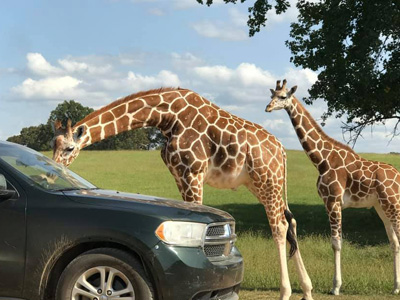In this photograph, two giraffes are captured in an outdoor, likely safari-style setting. The main focus is on a large giraffe bending down to the driver's side window of an older, green car, possibly a Dodge from the 80s, that sits in the lower left corner of the image. A person's hand is extended from the window, feeding the giraffe. Standing a little behind and to the right is a smaller giraffe, observing the scene. The background features a vast meadow with light greenish-yellow grass, and a few scattered trees in the distance with dark green foliage. A tree branch with hanging leaves drapes into the upper right corner of the image, all set against a backdrop of blue sky filled with large, puffy clouds. The car, slightly rusty and splattered with mud, is parked on a dirt road that cuts through this serene landscape.